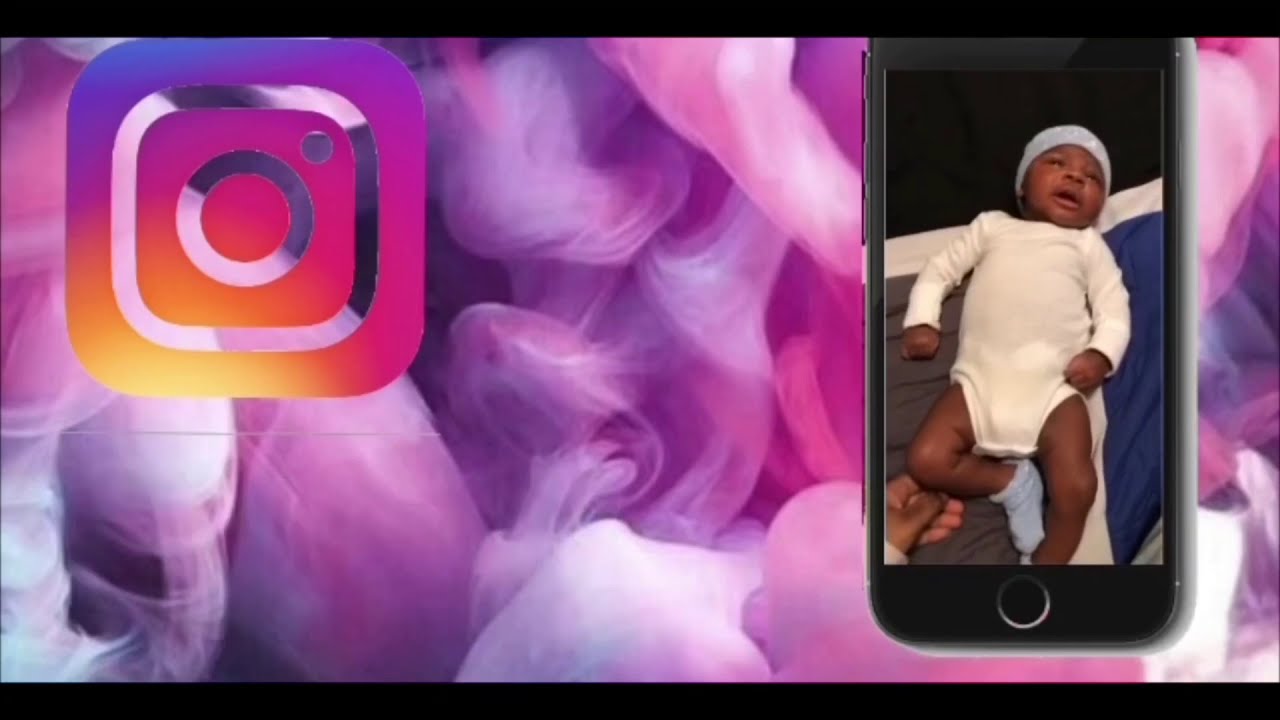The image is a detailed rectangular composition featuring two distinct elements. The background is a vivid swirl of pink smoke, reminiscent of cotton candy or cigarette smoke, creating a soft, dreamy atmosphere. In the upper left-hand corner of this background lies the Instagram app icon, notable for its colorful gradient transitioning from yellow and orange to dark purple and pink.

Dominating the right side of the image is a smartphone with a black bezel and a white circle button at the bottom, appearing to hover against the smoky backdrop. The phone seems to be encased in a clear protective cover. Displayed on the phone's screen is a photograph of a young baby with very dark skin. The baby is dressed in a long-sleeved white onesie and a light blue skull cap, with one foot drawn up revealing a grayish-blue sock, while the other leg is stretched out, making the second foot less visible.

The baby lies on a surface with a color scheme of gray, blue, and white. Behind the baby’s head is a solid black background, providing a stark contrast to the colorful surroundings. Near the baby's bent elbow, there’s a visible hand touching the edge of the baby’s knee, adding a gently interactive element to the scene. Thin black borders frame the top and bottom edges of the image, further enhancing its visual structure.